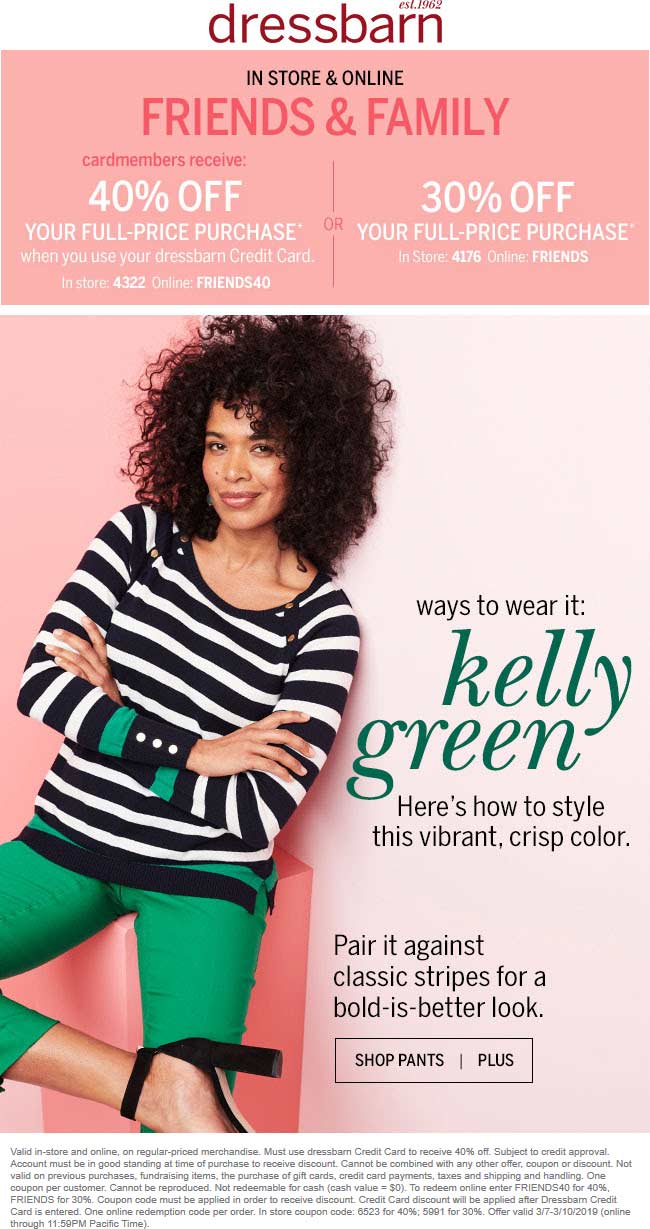This is an ad screenshot for Dress Barn. At the top, in dark red lowercase letters, it reads "Dress Barn established in 1962." Just below, there is a wide pink banner with text reading "in store and online friends and family." Below the banner, the content is divided into two sections by two vertical lines with the word "or" in the center. 

- On the left side, it says: "Card members receive 40% off your full-price purchase when you use your Dress Barn credit card. In store: 4322. Online: FRIENDS40."
- On the right side, it reads: "30% off your full-price purchase. In store: 4176. Online: FRIENDS."

Beneath the pink banner is a vertically-oriented rectangular image. The image portrays a dark-haired, dark-skinned woman leaning towards the right with her arms crossed. She is wearing a stylish black and white striped t-shirt, which features a green stripe just above the cuffs and three white buttons on the cuffs. The woman is also sporting tight green capri pants. Her right leg is bent at the knee with her right foot and ankle crossed over her left thigh. Completing her chic outfit are black heel sandals with an ankle strap.